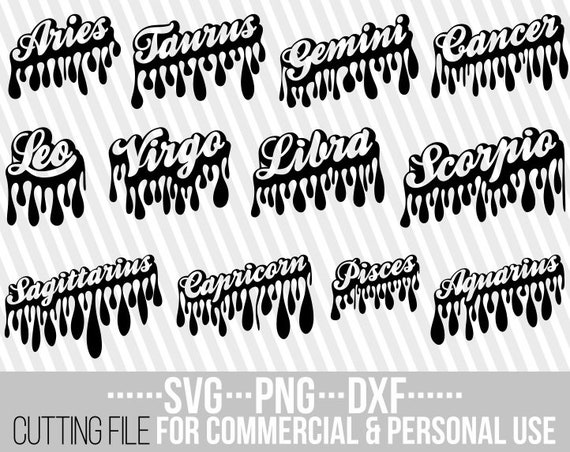The image is an advertisement for a cutting file that can be used for both commercial and personal purposes, available in SVG, PNG, and DXF formats. Displayed centrally are the names of the astrological signs, arranged from Aries at the top left to Aquarius at the bottom right, with four signs per line across three lines. The signs are depicted in a bold, script font predominantly in black, with a striking drop shadow effect that creates the appearance of paint dripping beneath each word. The background features diagonal, alternating gray and white lines running from the top left to the bottom right, enhancing the visual appeal. At the bottom of the image, a gray border displays several dots followed by the text: "cutting file" in black, "SVG," "PNG," and "DXF" separated by dots in white, and concluding with "for commercial and personal use" in black. This cohesive design effectively communicates the available formats and intended uses of the cutting file, accentuated by its monochromatic color scheme.